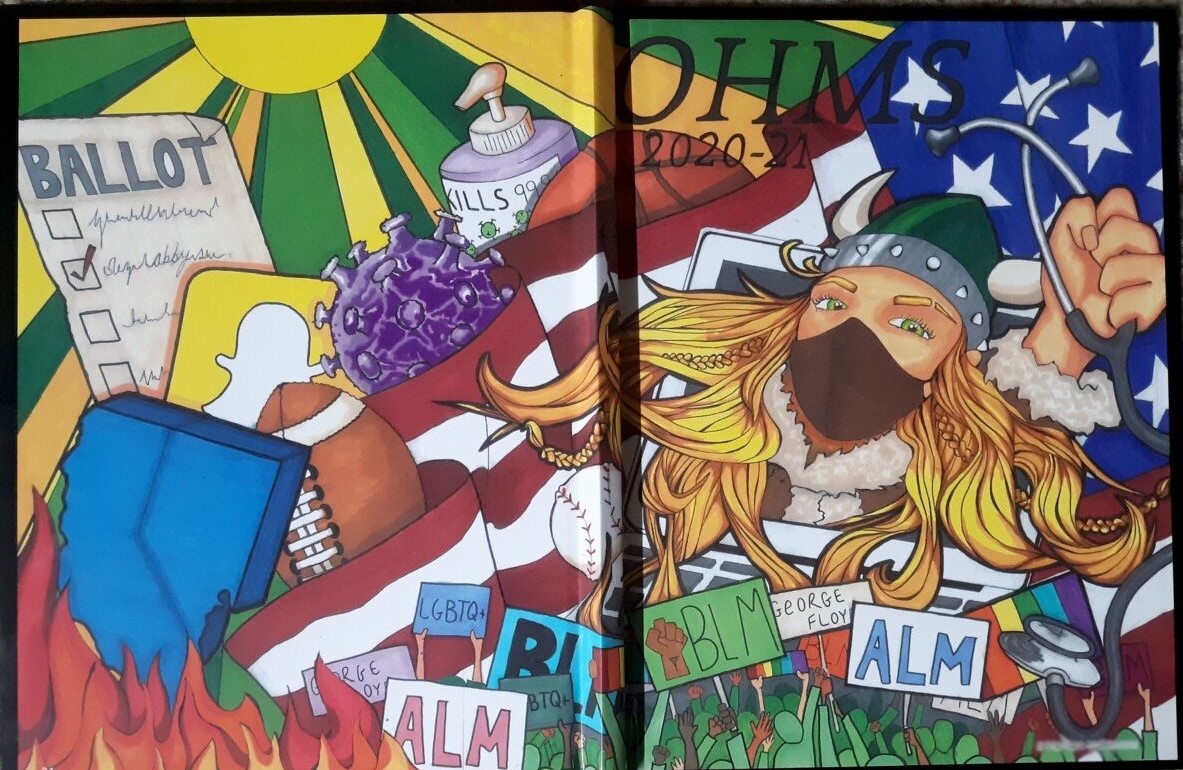The illustration titled "OHMS 2020-2021" appears as a split-page design, resembling a book with a crease down the center. The left page features a vibrant sun with yellow, orange, and green rays. Surrounding the sun are contemporary symbols such as the Snapchat logo, a detailed rendering of the coronavirus, and a lavender bottle of hand sanitizer labeled "kills 99% of germs." A ballot with a checkmark signifies voting, next to which are a football and a blue rectangle. At the bottom left corner, flames are depicted, adding a sense of urgency and intensity.

On the right page, a striking Viking woman stands central, decked in a dark green helmet with horns, a brown fur coat, and a black face mask. She holds a stethoscope in her left hand, symbolizing the medical community. Her long blonde hair flows dramatically across the scene, blending into the left side of the page. The background boasts a prominent American flag. Below her, various green-tinged individuals raise protest signs advocating for ALM, George Floyd, BLM, and LGBTQ+ rights. A colorful Pride flag is noticeable among the crowd, tying in with the broader themes of equality and justice.